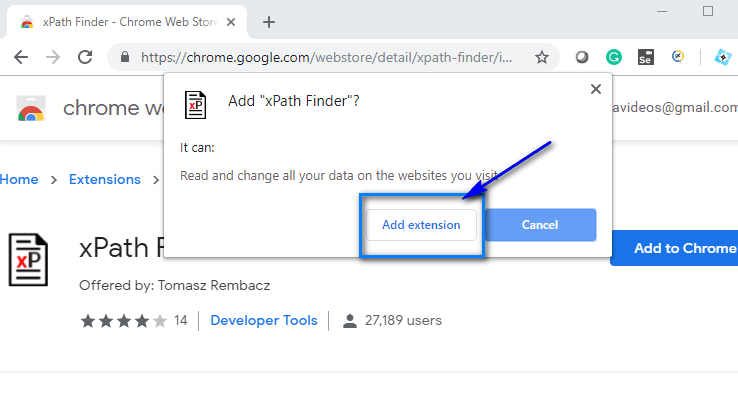A person is interacting with a Chrome browser window, specifically on the page for adding a browser extension named "XPath Finder" from the Chrome Web Store. The browser address bar shows chrome.google.com/webstore/detail, indicating they've navigated to the extension's detail page. The screen displays a pop-up that asks for permission to add the "XPath Finder" extension, which states that it can read and change all data on websites visited. The pop-up offers two buttons: "Add extension" and "Cancel."

In the background, details about the extension are visible, such as its name—offered by Tomas Rembaks—along with a 4-star rating based on 14 reviews, categorization under developer tools, and usage by 27,189 users. Notably, the "Add extension" button has a prominent purple arrow pointing towards it, encased within a large blue rectangle featuring an exaggerated drop shadow, making it stand out significantly. The "Cancel" button is located to the right of the "Add extension" button. Below the pop-up, there's a "Add to Chrome" button, which presumably, once clicked, triggered the appearance of the permission pop-up. The design of the pop-up window itself is minimalistic, with a white background and a thin drop shadow on three sides (right, left, and bottom) and a fine pixel line on the top edge.